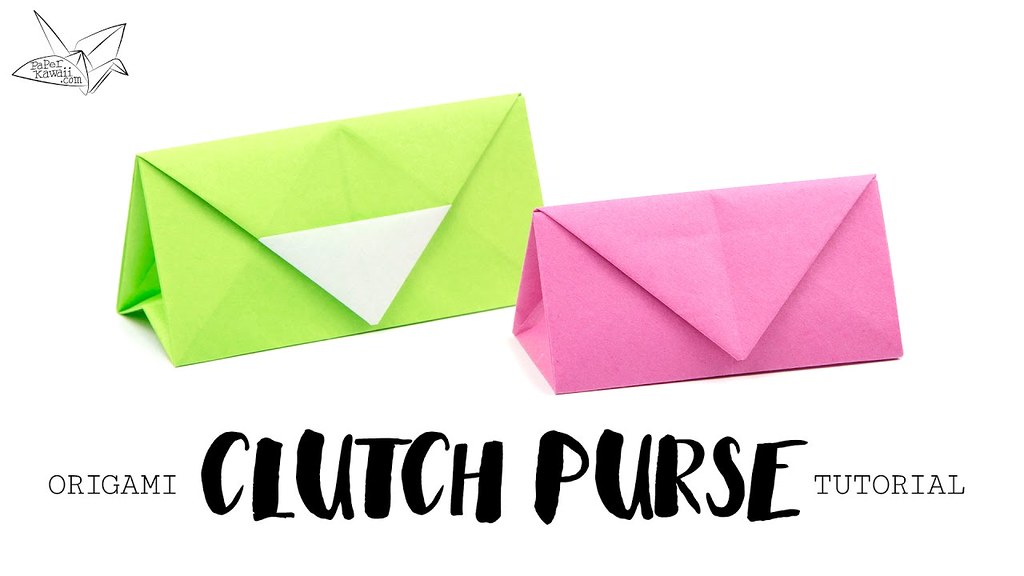This image features a detailed illustration titled "Origami Clutch Purse Tutorial," prominently displayed at the bottom. It showcases two striking origami purses crafted from paper using intricate folding techniques. In the upper left corner, the website pawperkawaii.com is marked on a small origami bird.

The purse on the left is a vibrant lime green with a contrasting white point where the clasp would be. This purse has a slightly larger, envelope-like 3D design. To its right, the second purse is a smaller, bright fuchsia pink, also resembling an envelope. Both purses are visually appealing, notable for their bold colors and precise craftsmanship. While their practicality might be limited due to their paper construction, they make for an attractive and engaging project, ideal for enthusiasts of origami and arts and crafts.